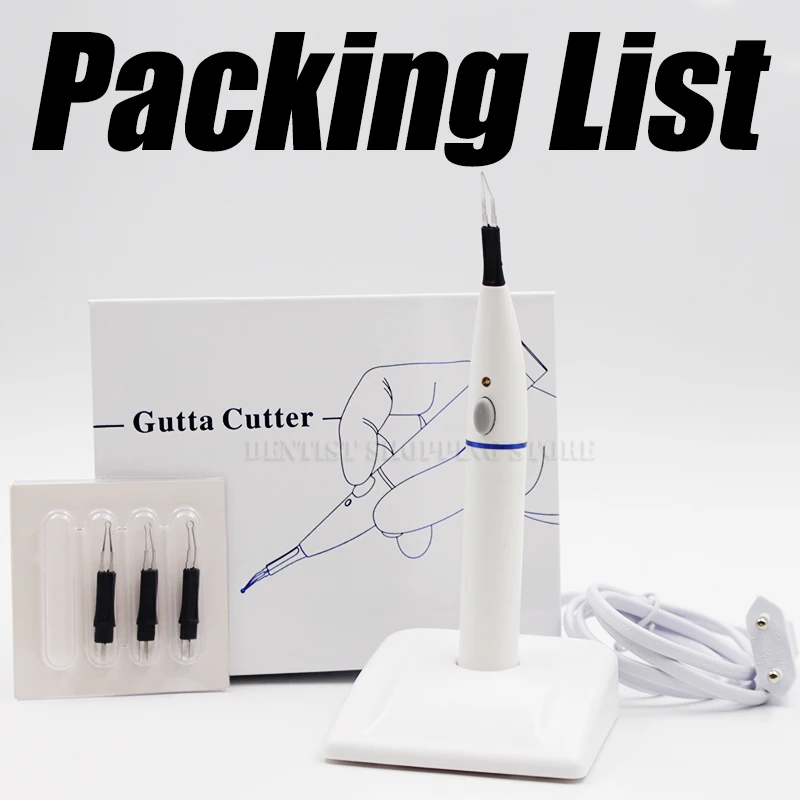The image showcases a dental cleaning device, referred to as a "gutta cutter," resembling an electric toothbrush but designed with a sharp plastic tip. This white device features a gray oblong-shaped button and a small circular indicator, likely for a light. A blue band encircles its tubular midsection. The gutta cutter is positioned upright in a white base, which also functions as its charger.

At the image's upper section, the words "Packing List" appear against a light gray background. Accompanying the device are four extra tip attachments, with three still in a packet located at the bottom left and one inserted into the device. Additionally, a folded document labeled "gutta cutter" is visible, possibly including instructions, and there is a depiction of a person using the device by pressing its button. The bottom right corner shows a plug and wires necessary for charging.